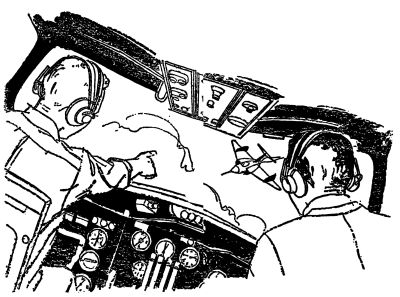This black-and-white hand drawing, possibly created with a pen or marker, depicts two male pilots inside the cockpit of their airplane, replete with an array of instrument panels, gauges, switches, and levers. Both pilots have short hair and wear headphones. They are gazing out of the cockpit's front window, with the pilot on the left pointing with his right hand towards a smaller aircraft in the distance, which could be a fighter jet or an older-style plane, flying above a cloud. The drawing captures several intricate details inside the cockpit, including various buttons, knobs, and other instruments located at knee height and overhead. Though devoid of text, the image conveys a scene filled with action and technical details, set against a backdrop of clouds in the sky.